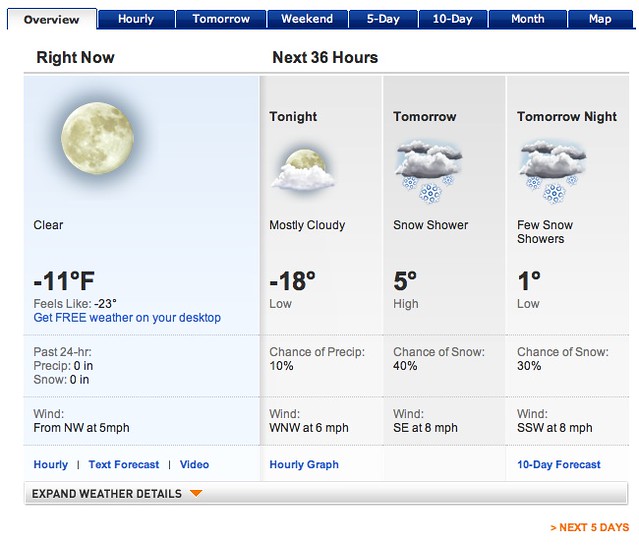The image is a screenshot taken in landscape mode, likely from a laptop, showcasing a weather application. In the bottom right-hand corner, there is an interactive orange button labeled "Next 5 Days," allowing users to access further weather information. On the bottom left, bold black text reads "Expand Weather Details," accompanied by a downward-pointing orange triangle. The lower section of the image features a white area.

The main content of the screenshot centers around weather information. In the upper left corner, the selected tab is "Overview," highlighted in white, while other tabs— "Hourly," "Tomorrow," "Weekend," "5 Day," "10 Day," "Month," and "Map"—are displayed in blue with white font, indicating they are not selected.

The next row divides the weather details into two columns. The left column displays the current weather with a large moon icon, indicating clear conditions with a temperature of -11°F, feeling like -23°F, and a prompt to "Get Free Weather on Your Desktop." Additional details include the past 24 hours' precipitation (0 inches) and snow (0 inches), and the wind coming from the northwest at 5 mph. Below this section, there is a blue text link for "Hourly Text Forecast Video."

The right section is organized into three columns, labeled "Tonight," "Tomorrow," and "Tomorrow Night." Each column features weather icons: a cloudy moon for "Tonight," and snowy clouds for both "Tomorrow" and "Tomorrow Night," reflecting expected weather conditions.